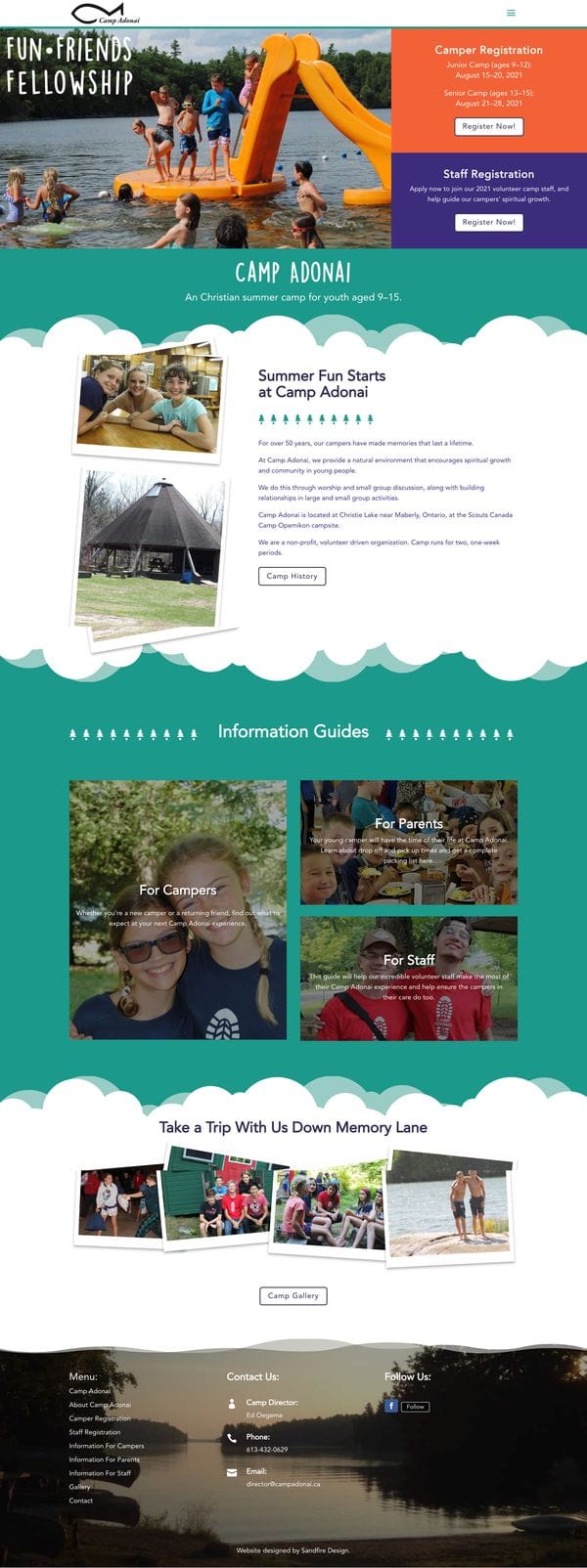The brochure displayed on the mobile device prominently features a vertically long layout. At the top left corner, the title "Fun, Friends, Fellowship" is written in a white, animated font. Beneath the title, there is a vibrant image of twelve children enjoying an orange inflatable slide in the middle of a picturesque lake surrounded by trees. Some kids are in the water while others remain on the slide's platform.

Adjacent to the image, the brochure provides options for "Camper Registration" and "Staff Registration." Directly below this section, another area introduces "Camp Adonai," detailing it as a Christian summer camp for youth aged 9 to 15. The tagline "Summer fun starts at Camp Adonai" is clearly visible, although the descriptive text is too small to read easily. There's a clickable button to explore more about the camp's history.

Following this, the next section marked "Information Guide" offers specific guides categorized for campers, parents, and staff. Beneath this, the section titled "Take a Trip with Us Down Memory Lane" features a button linking to the camp gallery, allowing visitors to view photos from past events. At the very bottom, contact tabs provide information on how to reach the camp and navigational options through a menu bar.